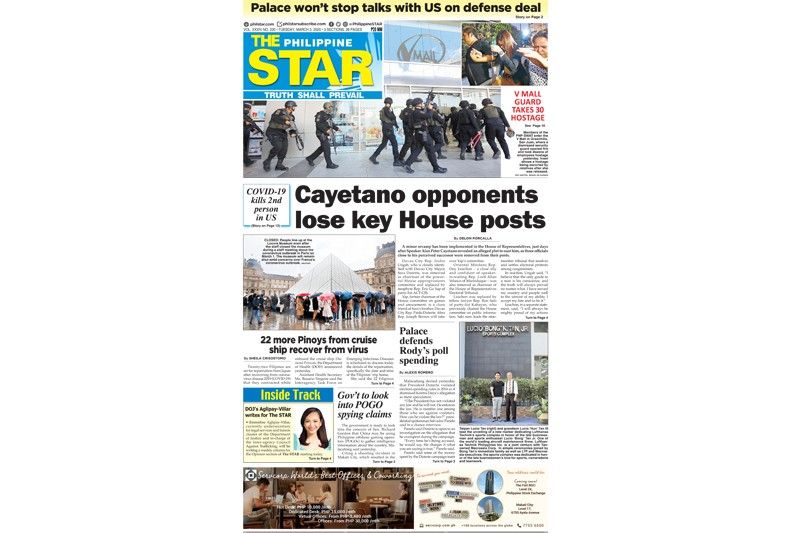A detailed caption for the provided image could be:

"A newspaper front page from The Philippines Star is featured prominently in the top left corner of the image, set against a vibrant blue background with striking yellow and white lettering. The title 'Star' is particularly noticeable in large, bold font. At the top of the page, a yellow banner contains the headline 'Palace won't stop talks with U.S. on defense deal' in bold black letters. 

The upper section of the front page showcases several images, including two photographs to the right of the star logo depicting people praying in front of a mall. Below these photographs, a wide banner image spans from left to right, showing a dramatic scene of military forces actively storming a mall. Adjacent to this, a red headline reads, 'V-Mail Guard takes 30 hostage.'

The main headline in bold black letters announces, 'COVID-19 kills second person in U.S.' To its right, against a white newspaper background, another headline states, 'Cayetano opponents lose key house posts.' On the left side of the newspaper, there is a picture showing people outdoors in the rain, identifiable by their open umbrellas, standing in front of a white triangular object.

Further down, the left section of the page declares, '22 more Pinoys from cruise ship recover from virus,' while the right section presents, 'Palace defends roadies poll spending.' Continuing downward, in the next section, yellow lettering on a blue background reads, 'Inside Track,’ accompanied by a picture of a young woman, suggesting an op-ed or commentary piece. To the right, a headline declares, 'Government to look into POGO spying claims.' Finally, at the very bottom of the page, there are two additional images likely pertaining to advertisements.'"